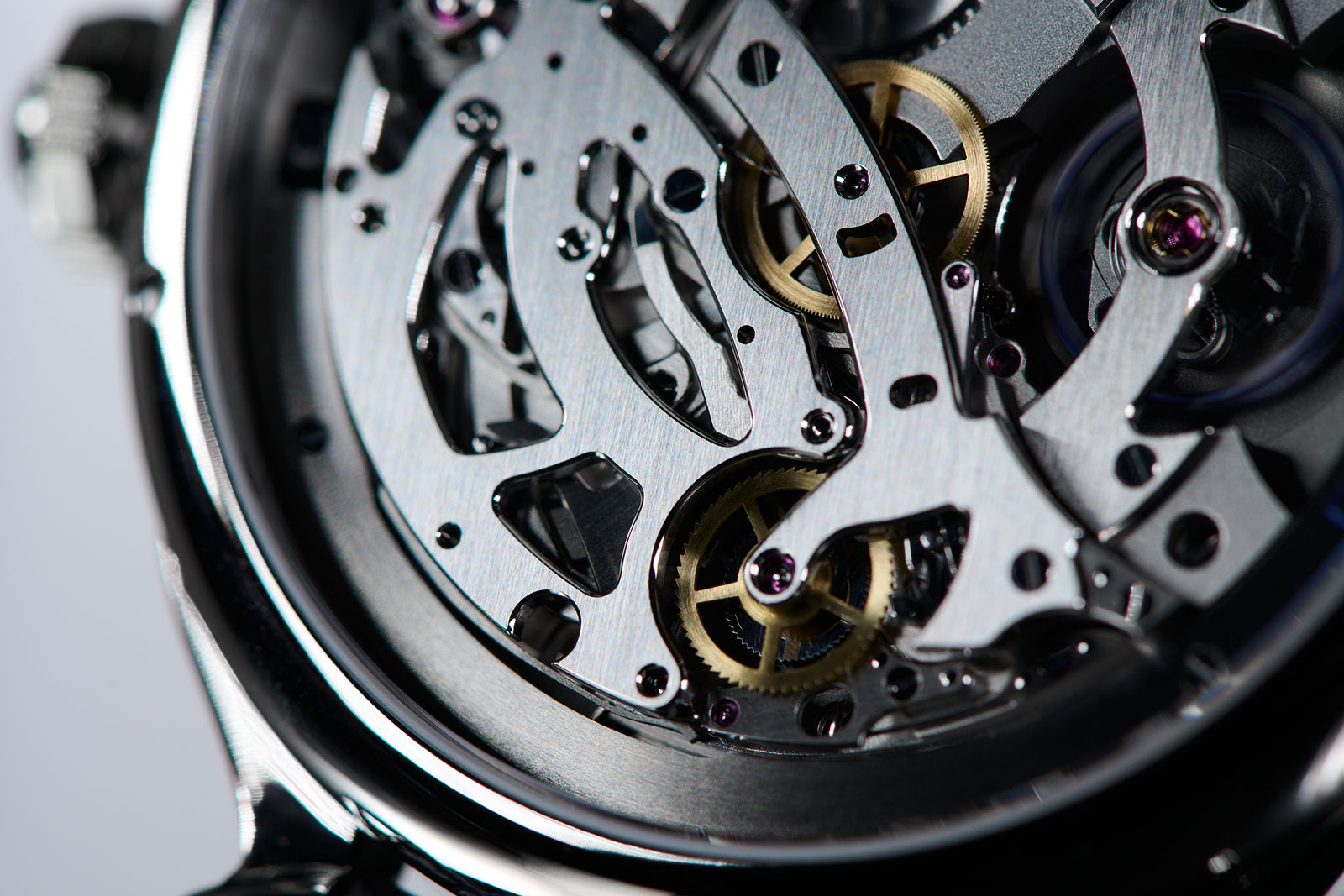The close-up photograph vividly captures the intricate inner workings of a wristwatch. Dominating the image is the round, dark slate brown watch head, which fills about seven-eighths of the frame, leaving a sliver of white background visible on the left. In the foreground, the outer circumference features a prominent knob used to reset the dials, affirming its identity as a wristwatch. The central focus is the elaborate array of gears housed within the watch, including several silver metal gears with tiny silver screws and holes. Notably positioned towards the middle are two gold gears, one atop the other, separated by a couple of centimeters, adding a striking contrast to the overall industrial design. To the right, a distinct black wheel, presumably another gear, is adorned with an almost purple screw, adding a subtle pop of color to the meticulously crafted mechanical ensemble. Encompassing these internal components is a silver ring that rounds off the watch head's sophisticated appearance.